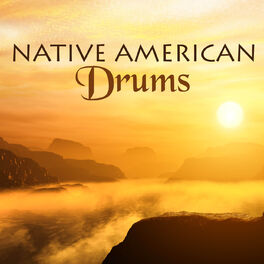This image, likely an album cover for a musical album, prominently features the title "Native American Drums" in black, with "drums" slightly darker in brown text. The background illustration captures a breathtaking canyon landscape, reminiscent of the Grand Canyon, with jagged, blackish-brown rock formations in the foreground. The scene transitions into a misty or foggy valley below, possibly the tops of clouds. In the background, more brown and black hills or mesas stretch across the image. Dominating the sky is an intense sunset, with vibrant hues of orange and yellow, casting a warm glow over the entire scene. The sun is positioned low on the right side, indicating late evening. The overall layout and imagery suggest this is indeed an evocative album cover, aiming to convey the raw natural beauty and the cultural essence of Native American drum music.